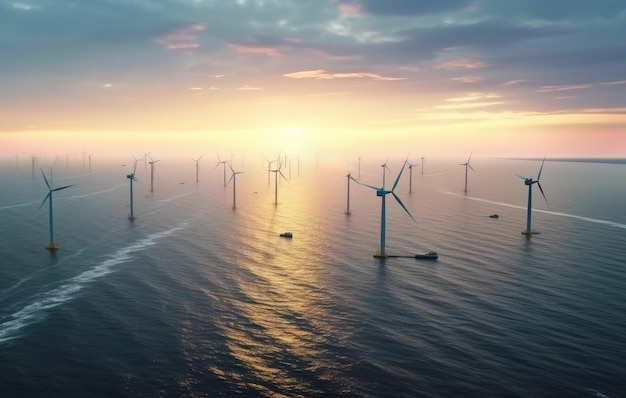This image captures a stunning sunset over a vast expanse of calm, dark blue water, likely from an ocean. The sky is painted with dark blue and gray clouds tinged with vibrant pinks and yellows, reflecting the setting sun's hues onto the water's surface. Despite the diffused bright light from the sun, visible along the horizon, one cannot discern its exact shape. Standing tall amidst the water, numerous wind turbines are scattered across the scene, with around twenty of them appearing to harness the wind's power. These turbines have thin, elongated frames with blades that point outwards, resembling arrows. Four turbines are distinctly visible, while the others fade into the background, blending with the blurred horizon. Small vessels or boats can also be spotted near these structures, adding a dynamic yet serene touch to the overall landscape. The image has a slightly surreal quality, making it seem almost computer-generated.